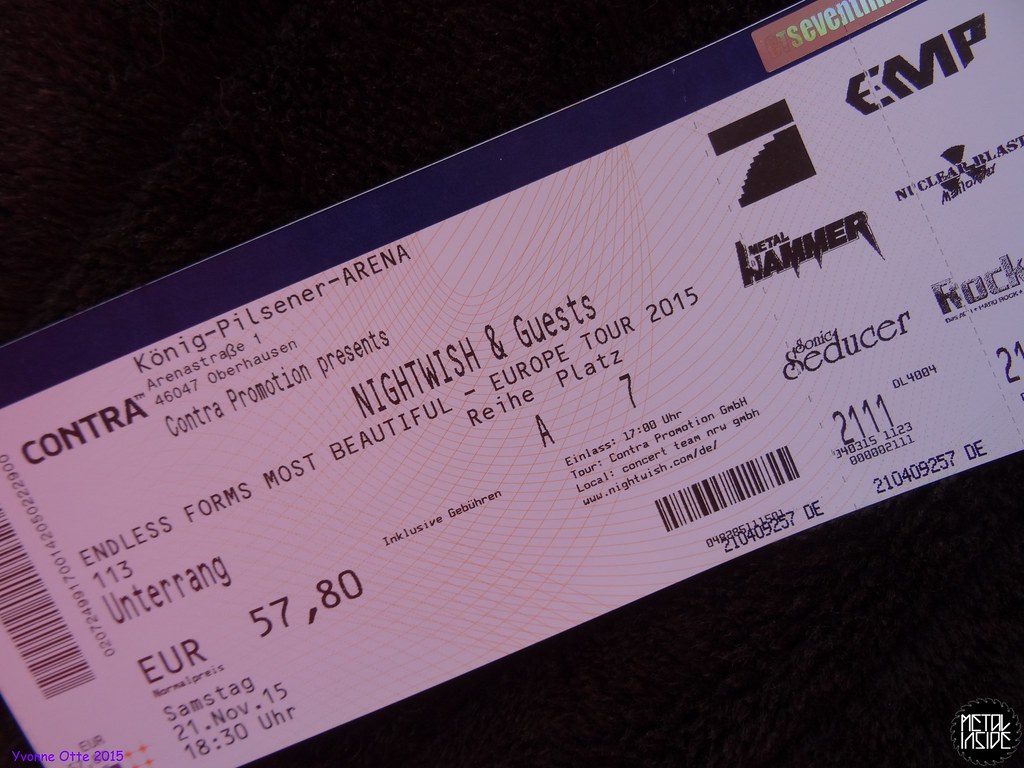This close-up image features a detailed view of an admission ticket for a concert event. The ticket prominently displays "Koenig Pilsner Arena" and details the event as "Contra Promotion presents Nightwish and Guests." The tour title is "Endless Forms Most Beautiful Europe Tour 2015." Additional information includes the event date and time: "Samstag, 21 November 15, 18:30 U.H.R." The ticket is priced at "57,80 Euro" and features a pink pattern with a blue section at the top. Notable elements include several barcodes, promotional logos on the right, and unique text such as "metal inside" in stylized letters. The ticket retains its stub and is designed for a concert or major event, potentially in Denmark.